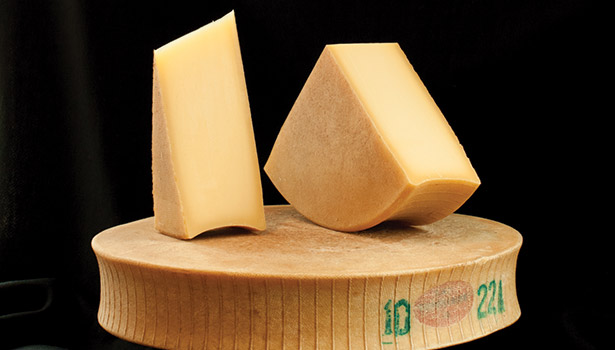The image features a detailed arrangement of three cheeses set against a completely black background. At the foundation, there's a substantial cheese wheel, characterized by its round form and vertical lines encircling the sides. This cheese wheel has green stamps displaying the numbers "10" and possibly "22-1" or "22-4," though the latter is difficult to read. A faded red circle label sits nearby on the wheel. The cheese wheel's exterior is brown with a tan top and reveals a white interior where it's been sliced. 

Positioned atop this wheel are two cheese slices. One is wedge-shaped reminiscent of a cheesecake slice, upright and with a firm rind, while the other slice resembles a larger cheesecake slice, also positioned upright and slightly tilting like a rocking chair. Both slices are light in color, suggesting a relatively mild cheese. In the left section of the image, a faint lighter shade of black interrupts the otherwise solid black background.